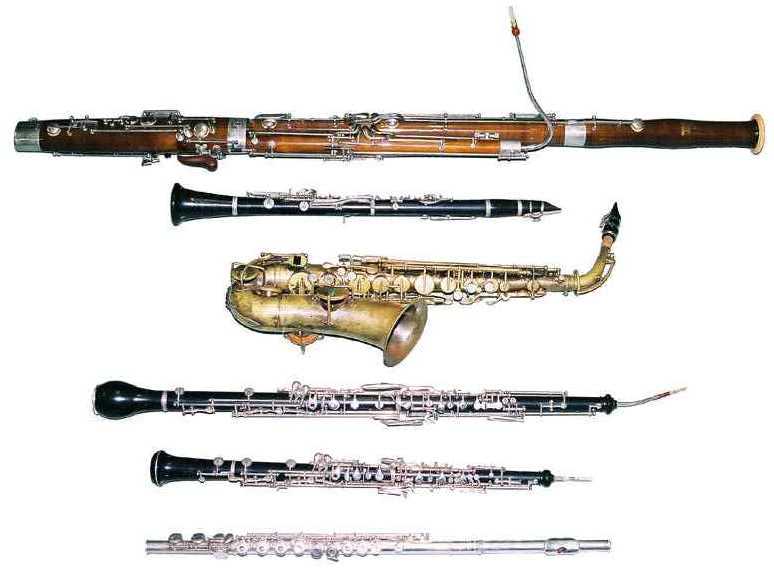The image features six different musical instruments arranged horizontally against a white background. At the top is a bassoon, characterized by its long cylindrical shape and brownish color that darkens towards the top. It includes a metal mouthpiece extension with a reed projecting upward and to the right. Below the bassoon is a black clarinet with silver buttons, oriented with its reed pointing down. The middle instrument is a golden saxophone, with its worn-looking bell facing right and the reed pointing left. Underneath the saxophone, there are two other black instruments, likely various types of clarinets or oboes; one is slightly longer than the other and has a distinct bulb at the bottom. The last instrument is a long, shiny silver flute, identifiable by its buttons on the left side and mouthpiece on the right.